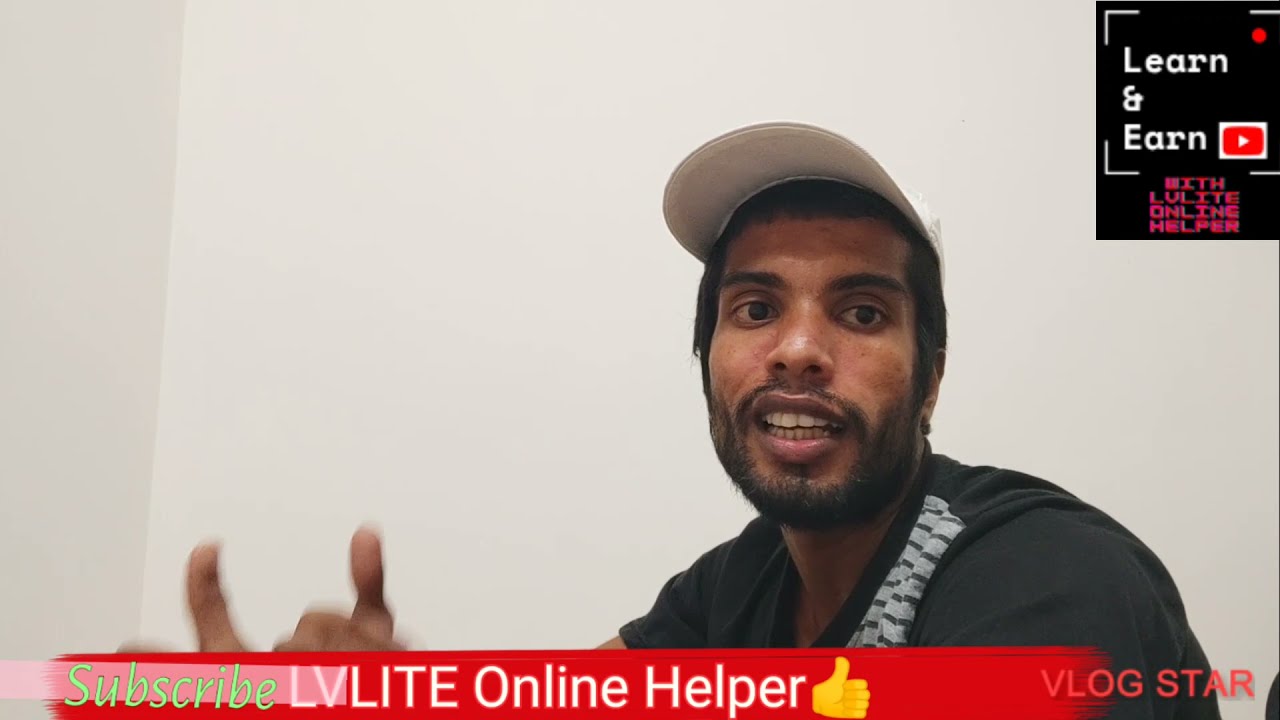The image appears to be a screen capture from a live YouTube video featuring a brown-skinned man centered in the frame, possibly of Indian descent, with a friendly smile and an engaged demeanor. He is wearing a white baseball cap, a black short-sleeve t-shirt, and has dark hair along with a short black beard and mustache. Both of his hands are in the frame, giving blurred thumbs-ups, indicating that the action was captured while in motion.

In the upper right corner of the screen, there is a small black box that reads "Learn and Earn" in white letters, alongside a red live indicator dot, and a red and white YouTube play button icon. At the bottom of the screen, a colorful banner features green text that says "Subscribe," white text that states "LV Lite Online Helper" with an accompanying thumbs-up emoji, and a red text label that reads "Vlog Star." The screenshot captures a vibrant mix of colors including off-white, brown, red, green, and gray, and suggests an indoor setting, possibly shot during the day. Overall, the image strongly indicates a live, engaging YouTube video aimed at providing educational or helpful content under the banner of "LV Lite Online Helper."